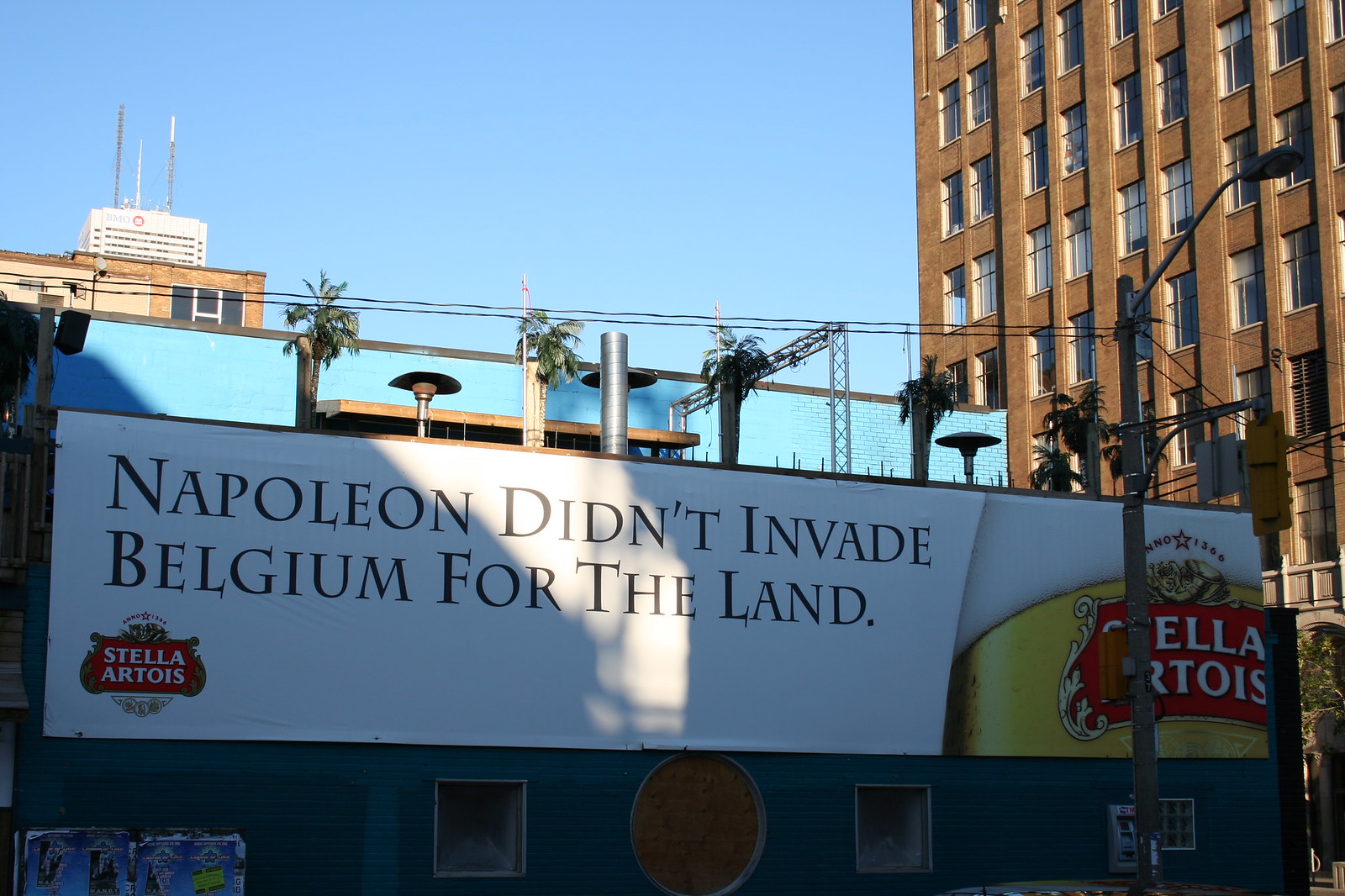This vibrant color photograph captures a unique urban scene. In the foreground stands a prominent sign with a white background and bold black text that reads, "Napoleon didn't invade Belgium for the land." Just below the text, on the left side, is the iconic red Stella Artois logo. Adjacent to this, on the right, is an appealing depiction of a glass of Stella Artois filled with golden beer, showcasing the brand's logo on the glass.

The setting includes the bottom edge of a bridge or the side of a building in shadow. The blue wall beneath it features square windows and a distinctive round wooden circle in the middle. To the right, a towering skyscraper dominates the skyline with its rectangular windows and brownish facade. Atop this building is an inviting dining area safeguarded by a thin black fence. The rooftop space has benches and round stools or tables scattered around, accompanied by lush plants with broad, thin leaves, adding a touch of greenery.

High above, a clear blue sky serves as the perfect backdrop, enhancing the contrasts and details of this captivating urban tableau.